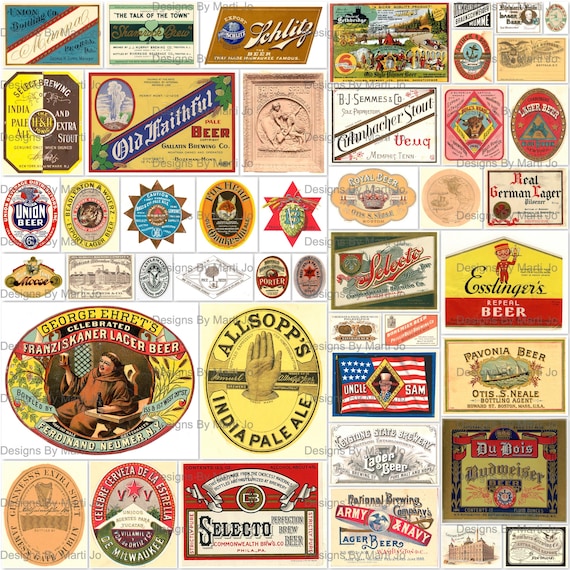The image depicts a meticulously arranged collage featuring 36 vintage beer labels organized in a grid of six rows and six columns, separated by gray lines. The labels showcase a diverse array of designs and colors. Notable labels include a blue rectangle with a white diagonal stripe and red borders, inscribed with the word "Union" in black writing; a white rectangle bordered in green with a black stripe across the middle; and a brown parallelogram with white letters and a blue circle. In the center, there's a yellow label depicting a hand and the words "Allsop's India Pale Ale," and nearby, a red star and an American flag label with "Uncle Sam." The collage features an eclectic mix of well-known and obscure beer brands, such as Schlitz, Budweiser, Old Faithful, Selecto, and George Earhart's, among others. The visual tapestry is completed with various shapes including circles, ovals, and rectangles, confirming the theme of old beer labels.